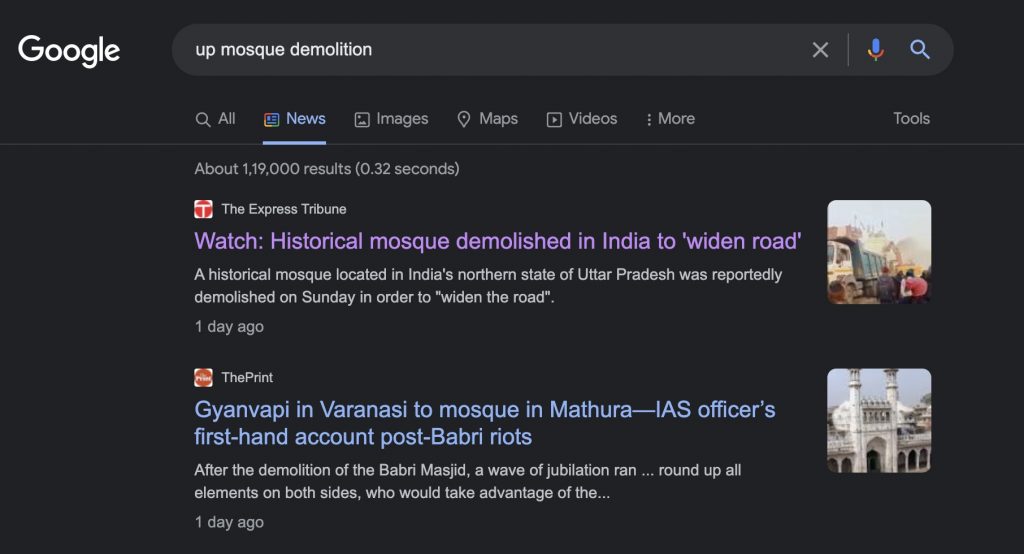The image features a black background displaying a Google search results page. In the top left corner, the Google logo is prominently visible in white with a capital "G" followed by "oogle." The search bar, which is dark gray, contains the text "mosque demolition" in white, accompanied by a white "X" for clearing the search, a blue microphone icon for voice search, and a blue magnifying glass icon for initiating the search.

Below the search bar, the navigation tabs are displayed: "All" in white, "News" in blue and underlined, "Images," "Maps," "Videos," "More," and "Tools" in white. Underneath this navigation menu, the page displays the search results information in white text, stating "About 119,000 results (0.32 seconds)."

The first search result is from Express Tribune and includes the headline, "Watch historical mosque demolition in India to widen road," also in white text. The snippet below provides more context, describing that a historical mosque located in India's northern state of Uttar Pradesh was reportedly demolished on Sunday to facilitate road widening. This article was posted one day ago.

Additionally, the page includes a blue link with the text "Gyanvapi Varanashi March mosque and Mthura district office's first hand account post property robbery riot," although the exact context and alignment of this text are less clear.